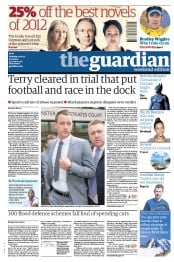This image features a page from either a tabloid or a newspaper, with various elements arranged strategically across it. At the top, there is a banner advertisement. The ad prominently displays "25% off" in bold maroon lettering, followed by "the best novels of 2012" in thinner maroon text. Beneath this header, black text provides additional details, with more bold maroon text at the bottom, separated by a black divider.

On the right side of the page, an ensemble of individuals is pictured: a blonde-haired woman, a gray-haired man in a tuxedo, and a dark-haired woman, laid out from left to right. Farther right, there's a sideways barcode. To the right of the barcode, a circular cutout features a man sporting a blue hat and a yellow shirt.

Below this, a dark blue header bears the text "The Guardian," with "The" in light blue and "Guardian" in contiguous white text of the same font. In the bottom right corner, some white text is present, though it’s indecipherable in this view.

Along the right margin, five distinct square areas showcase different features of the magazine. The first segment highlights Batman. The second square depicts a woman with dark hair styled in a bun, wearing a taupe-colored shirt. The third square appears to show a circular scenery, likely an ocean or sky in the background. The fourth box features a man in a dark blue shirt, while the final square has a dark blue background with some white text.

Dominating the left section of the page is the main story. The bold black headline reads: "Terry cleared in trial that put football and race in the dock."